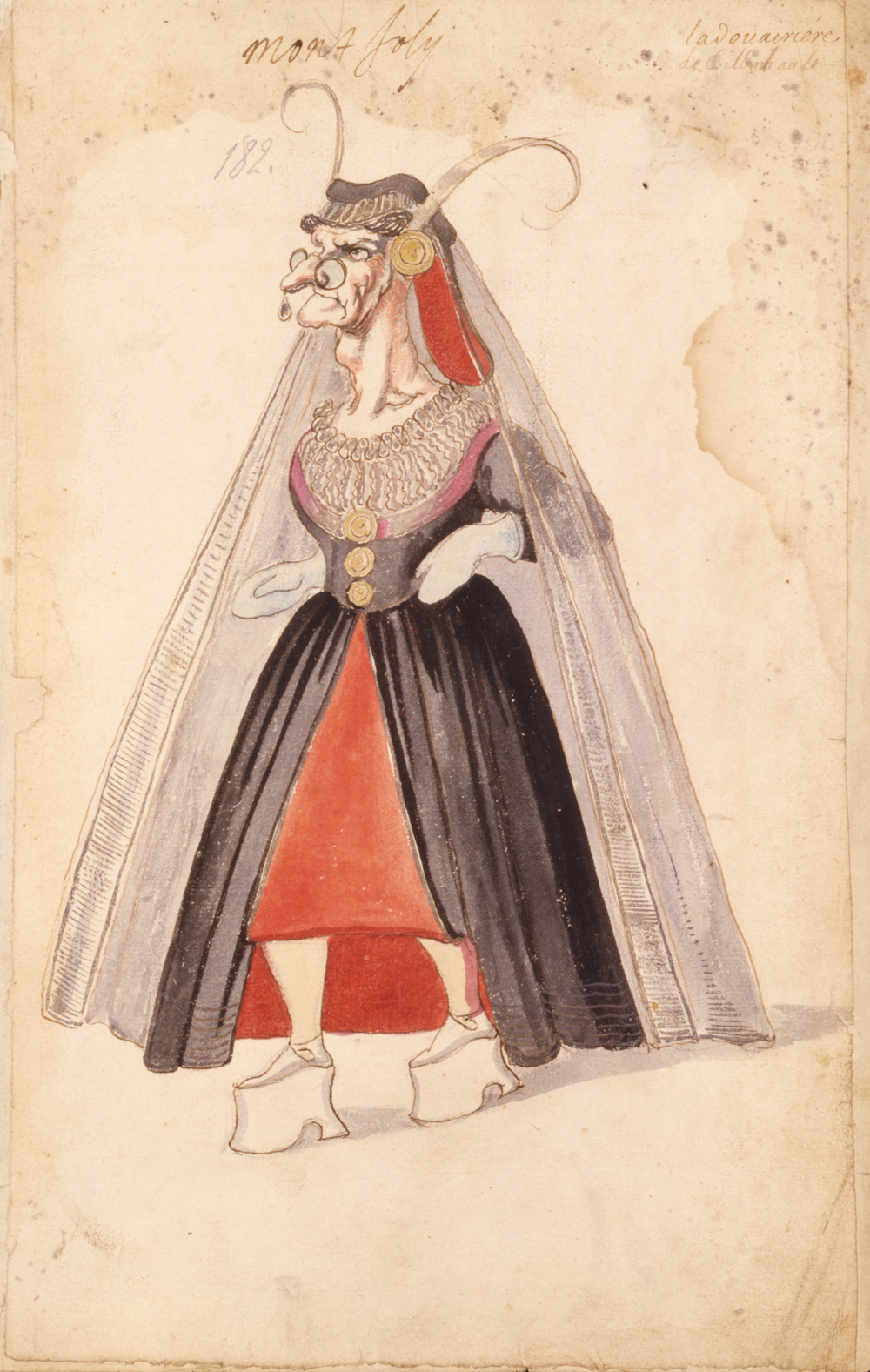The image is a detailed illustration on aged, light-brown parchment paper, depicting a hybrid creature with both human and animal characteristics. Central in the vertical rectangular frame is a woman-like figure standing in a three-quarter view and facing left. She is dressed in an elaborate vintage outfit featuring a tight black dress with a lace collar. The black dress splits open at the waist, revealing a red skirt underneath. The figure has white, gloveless hands—possibly suggested to be mittens—positioned at her waist, along with white platform shoes that are wide and tall.

Her neck is long and muscular, supporting a head with exaggerated old features, including a long hooked nose, a jutting chin, and prominent wrinkles. She wears black circular glasses perched on her nose and has slanted eyes that convey an angry expression. Atop her head, she dons a soft black cap from which long, curved horns emerge, resembling antelope or goat horns. Red hair is visible beneath the cap, and a translucent white veil cascades from her cap to the floor. There are faint, unreadable handwritten texts at the top of the image, which adds to the vintage feel of the illustration with subtle water stains.

Overall, this drawing intricately combines elements of human attire with fantastical and animalistic traits, set against an aged and worn backdrop.